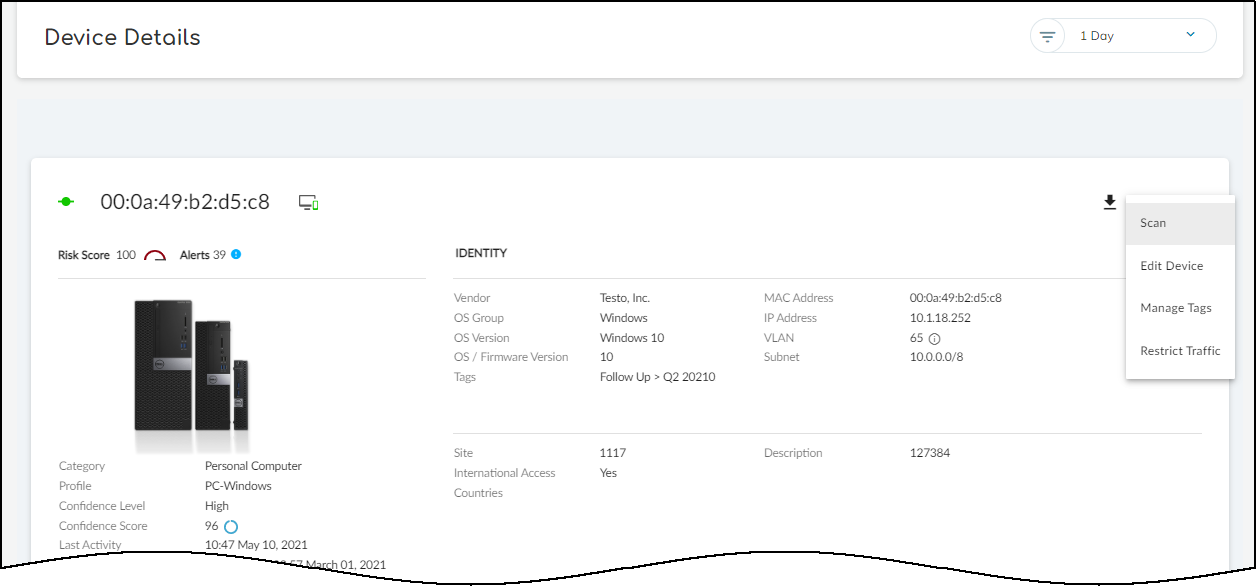This partial screenshot of a website features a light background and exhibits an unusual cropping style, with its bottom border forming a wavy line rather than a straight edge. At the top of the image, the heading "Device Details" is prominently displayed. Adjacent to this heading, a small box states "1 day" alongside an icon resembling an inverted pyramid composed of three lines, typically used to modify sorting or listing preferences.

Beneath this section, a gray area transitions into a white box that showcases an image of three Dell computers: a full-sized desktop, a mini tower, and a small form factor model, all arranged side by side in black. Below the image, descriptive text reads: 
- Category: Personal Computers
- Profile: PC, Windows
- Confidence Level: High
- Confidence Score: 96

To the right of this information, additional text provides further details about the computer's specifications, including the operating system and IP address.